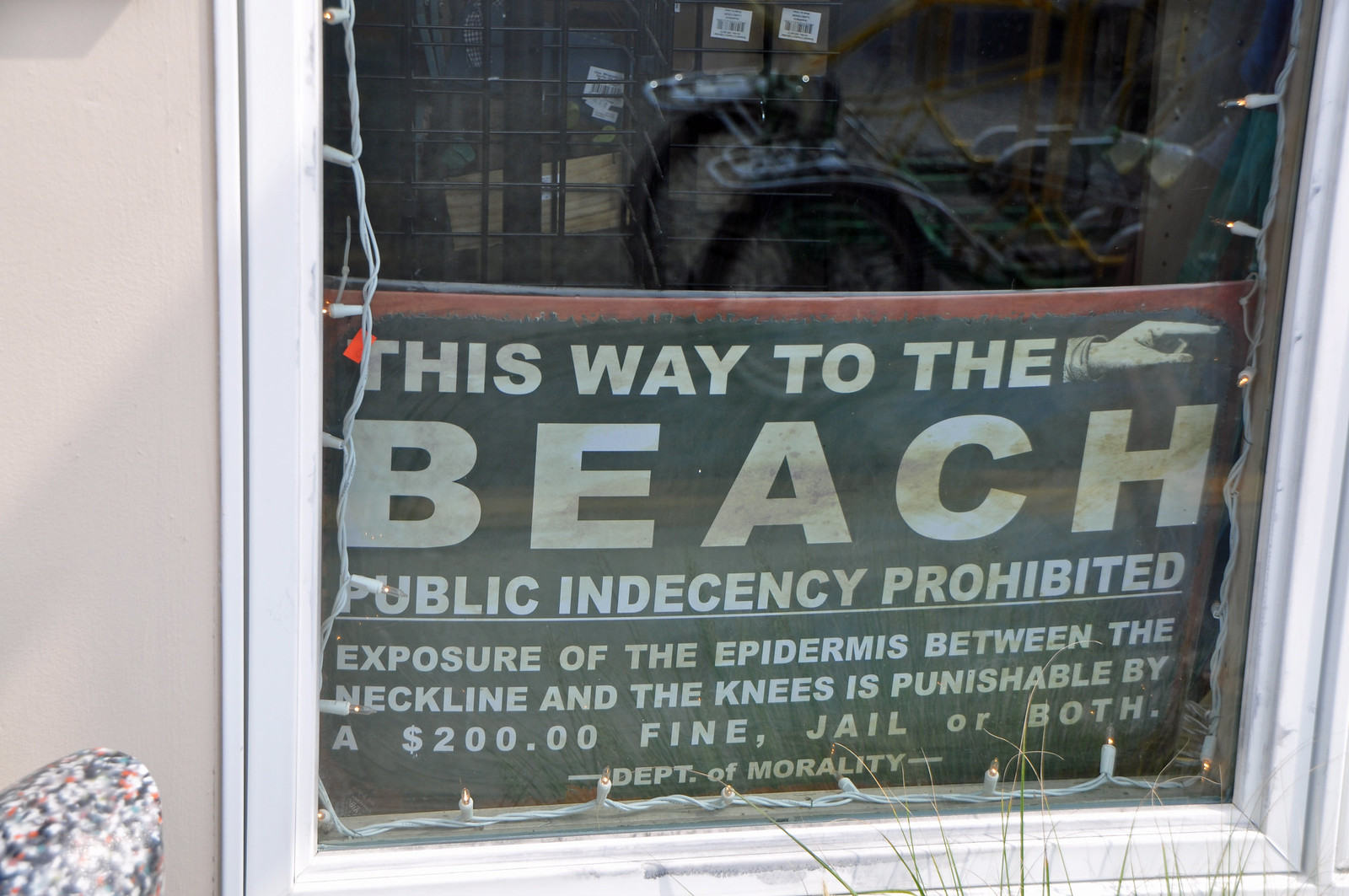The photograph features a wide, rectangular image capturing a window with a white frame, viewed from outside. The window appears situated in a beige-colored wall and contains white Christmas lights adorning its interior edges. Within the window, there is a dark green sign with a red border prominently displayed. The sign reads in bold off-white letters: "This Way to the Beach," accompanied by a graphic of a hand pointing to the left from the viewer's perspective. Below, it states, "Public indecency prohibited. Exposure of the epidermis between the neckline and the knees is punishable by a $200 fine, jail, or both." At the bottom, the sign is attributed to the "Department of Morality." A shiny, unidentifiable object is noted at the bottom left of the image, adding a subtle layer of curiosity to the scene. The photograph captures a mid-day outdoor setting near a building close to the beach.